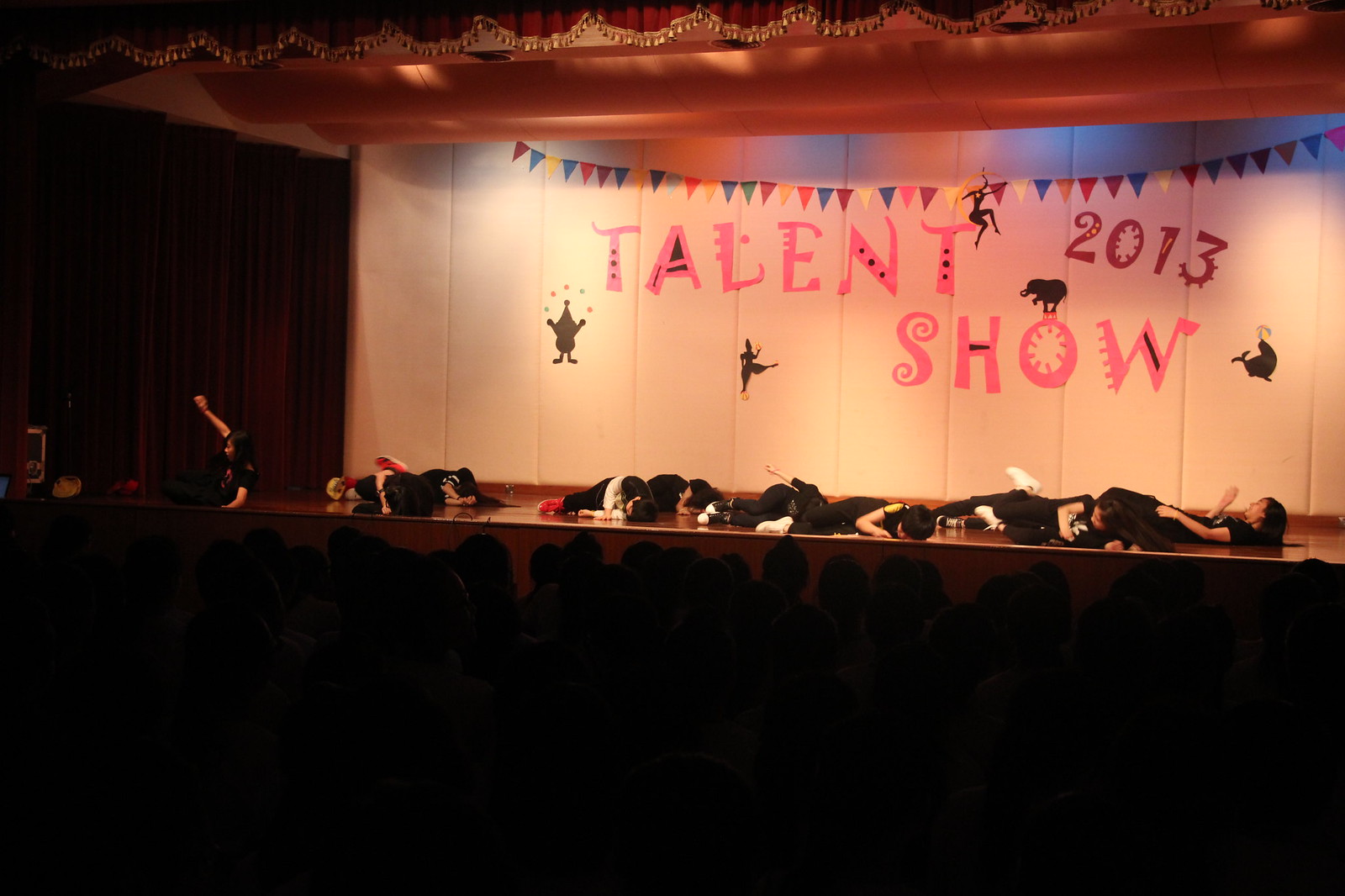The image depicts a dimly lit stage set for a talent show, prominently labeled "Talent Show 2013" in pink letters against a large white backdrop. Silhouettes of various figures, including a dancer, a whale, a seal, and a trapeze artist, are visible on the backdrop. The brightly lit stage contrasts with the darkened audience area, where only the heads of seated spectators can be faintly seen. The stage floor and top are brown, and there is a multicolored pennant, featuring hues of blue, red, yellow, and white, strung across the upper part of the backdrop. Above the backdrop, a tan ceiling with a canopy edge and recessed lighting completes the setting. On the stage, several performers dressed in black outfits with white accents, such as sneakers, are lying down, either at the beginning or the end of their act.